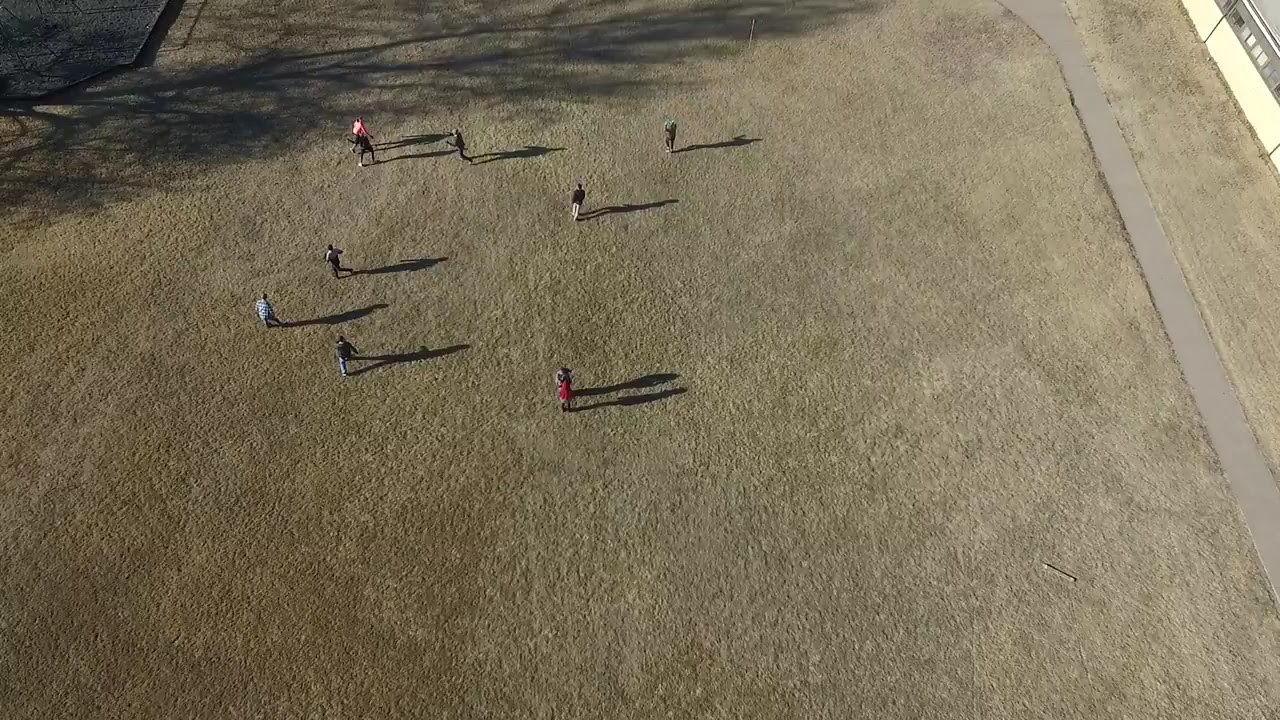This aerial photograph captures an expansive, open field with light brown grass, scattered with patches of green and dirt, suggesting a transitional season. At approximately 60 to 70 feet above ground level, the image reveals eight to possibly ten people dispersed across the field, their small size indicating the significant height from which the photo was taken. These individuals, whose genders are indiscernible, are concentrated more on the left side of the field, with their extended shadows adding to their numbers and complexity of positions. 

To the right side of the image, a narrow paved walkway runs parallel to the scene, adjacent to a slight grassy strip which leads to a structure with a yellow wall and windows situated in the upper right corner. The colors in the image primarily include variations of green, brown, gray, and yellow, with sporadic hints of red and pink from clothing. The scene lacks any visible sports equipment like goals or definitive field markings, although there might be a glimpse of someone kicking a soccer ball, suggesting some form of casual recreation or exercise. The photograph also features shadowy silhouettes of trees emanating from the upper left side, creating darker patches against the ground's lighter tones. The top left corner's distinct gray area could be an expanse of asphalt. Notably, the scene is void of any vehicles, animals, or textual elements, maintaining a purely natural and serene environment.